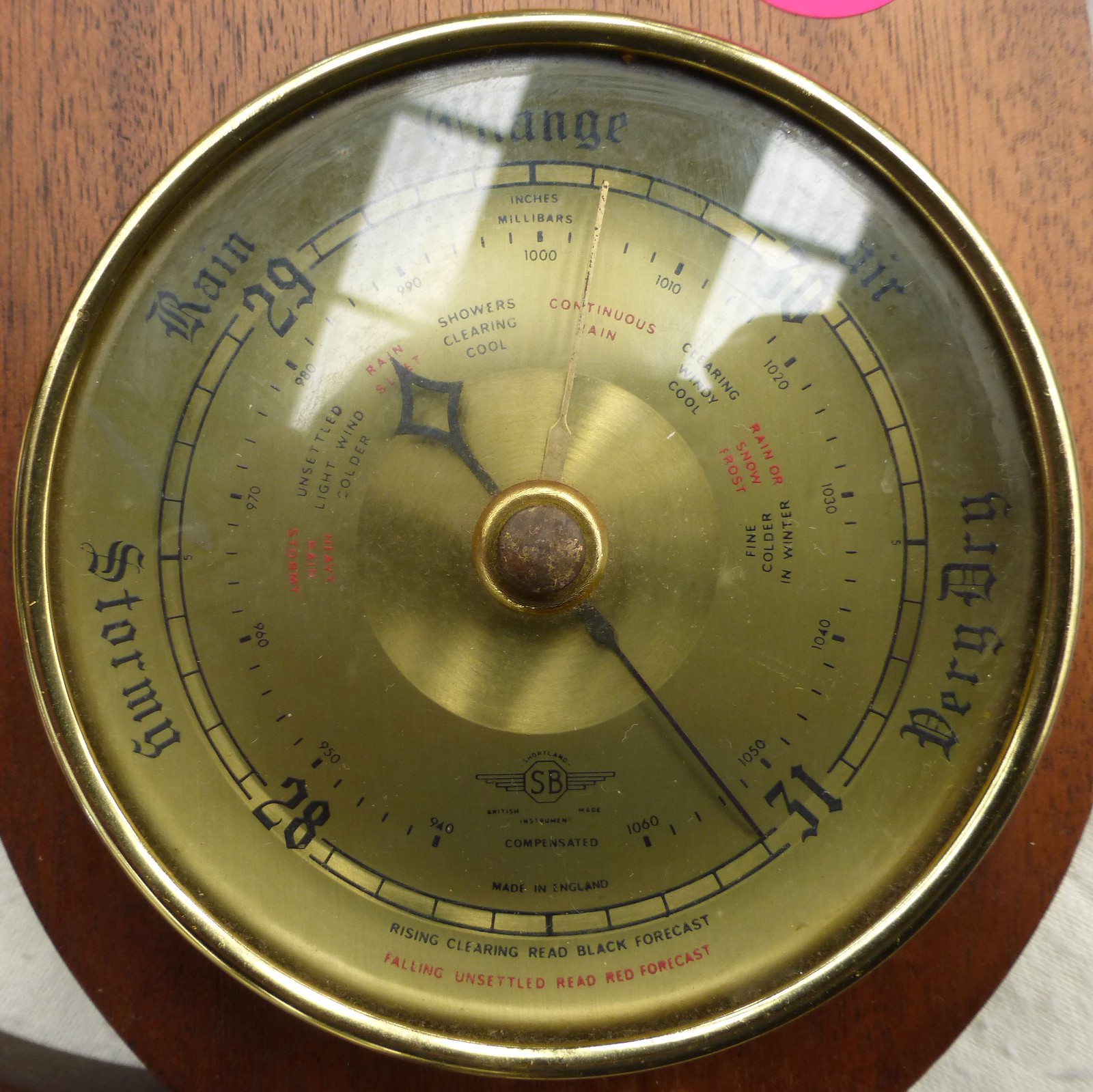This image captures a vintage, weathered barometer with a broad, golden metallic disc bordered by a wooden plaque and a glass covering. The barometer, possibly made in England, features a circular face with several concentric circles and a pair of clock-like hands. The outermost ring, marked with black and red text, delineates several weather conditions indicated by varying measurements. At the top center, partially obscured by glare, is the word "Change," followed by "Very Dry" around the one o'clock position and "Rising, Clearing, Read Black Forecast" at the bottom. Directly in red below this is the phrase "Falling Unsettled, Read Red Forecast." Other notable markings include "Air" near the top, "Stormy" at the eight o'clock position, and "Rain" between the ten and eleven o'clock positions. Surrounding these labels are numbers ranging from 28 to 31, with the hands pointing just past 31, suggesting very dry conditions. The inner dial, harder to read, indicates various states such as “Rain and Sleet” and “Continuous Rain” in red, interspersed with "Unsettled" and "Clearing, Windy, Cool" in black text. The face of the barometer intricately details various weather forecasts, and its aged patina and classical design hint at a bygone era of meteorological instrumentation.